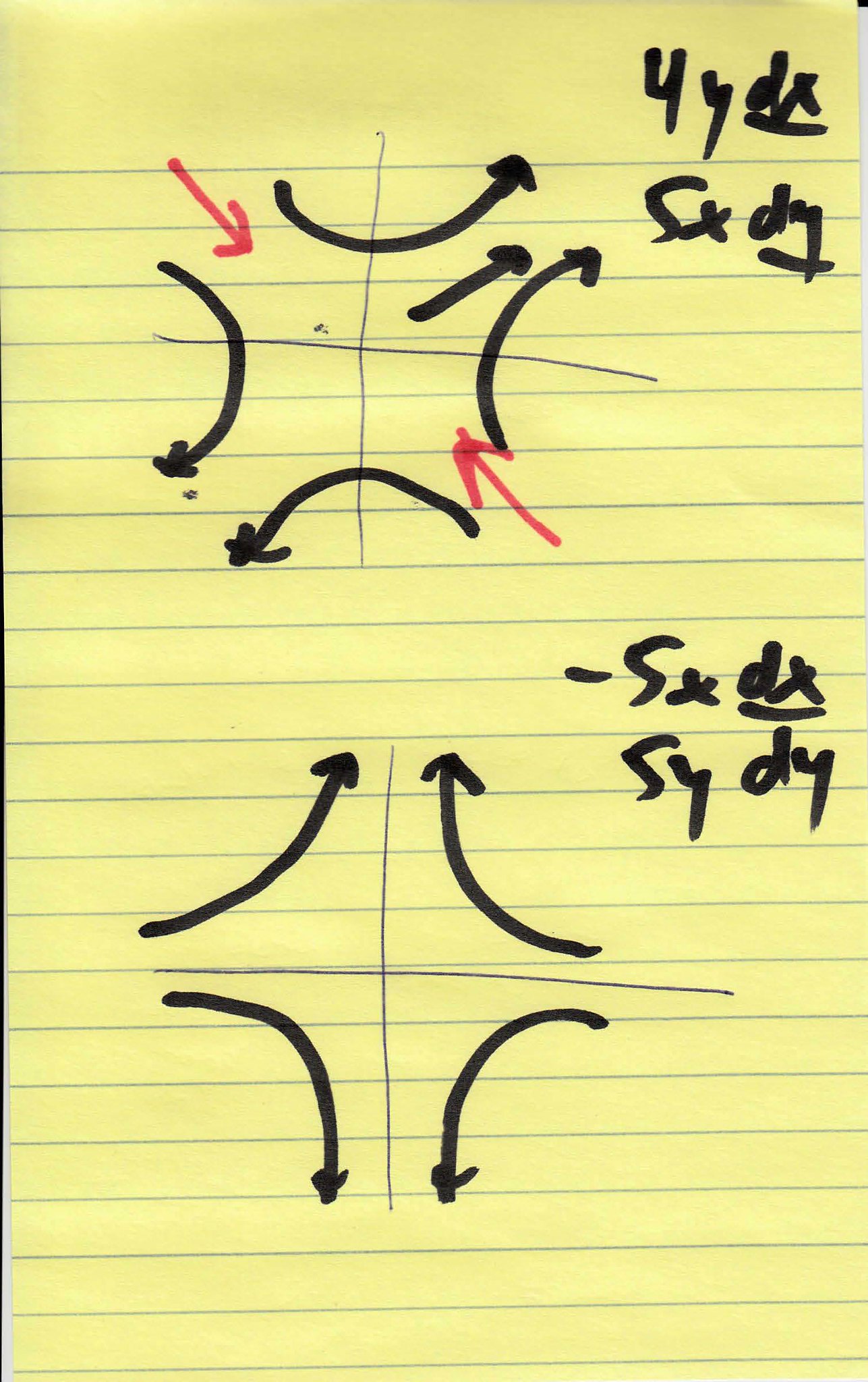A photograph depicts a yellowed piece of lined paper featuring handwritten notes and various markings. At the top right corner of the page, "4YDX" is written in black marker, underlined, followed by "CXDY" also underlined. Below these, an 'X' is drawn in pen. A series of black arrows cascade downwards, with a red arrow interspersed among them, and some of these arrows curve downward. Towards the middle of the page, "negative 5XDX" is written in black marker, underlined, and followed by "5YDY". Below this, an 'X' is drawn in blue pen. There are additional arrows pointing upwards and curving downward on the page, contributing to a complex and dynamic array of annotations.